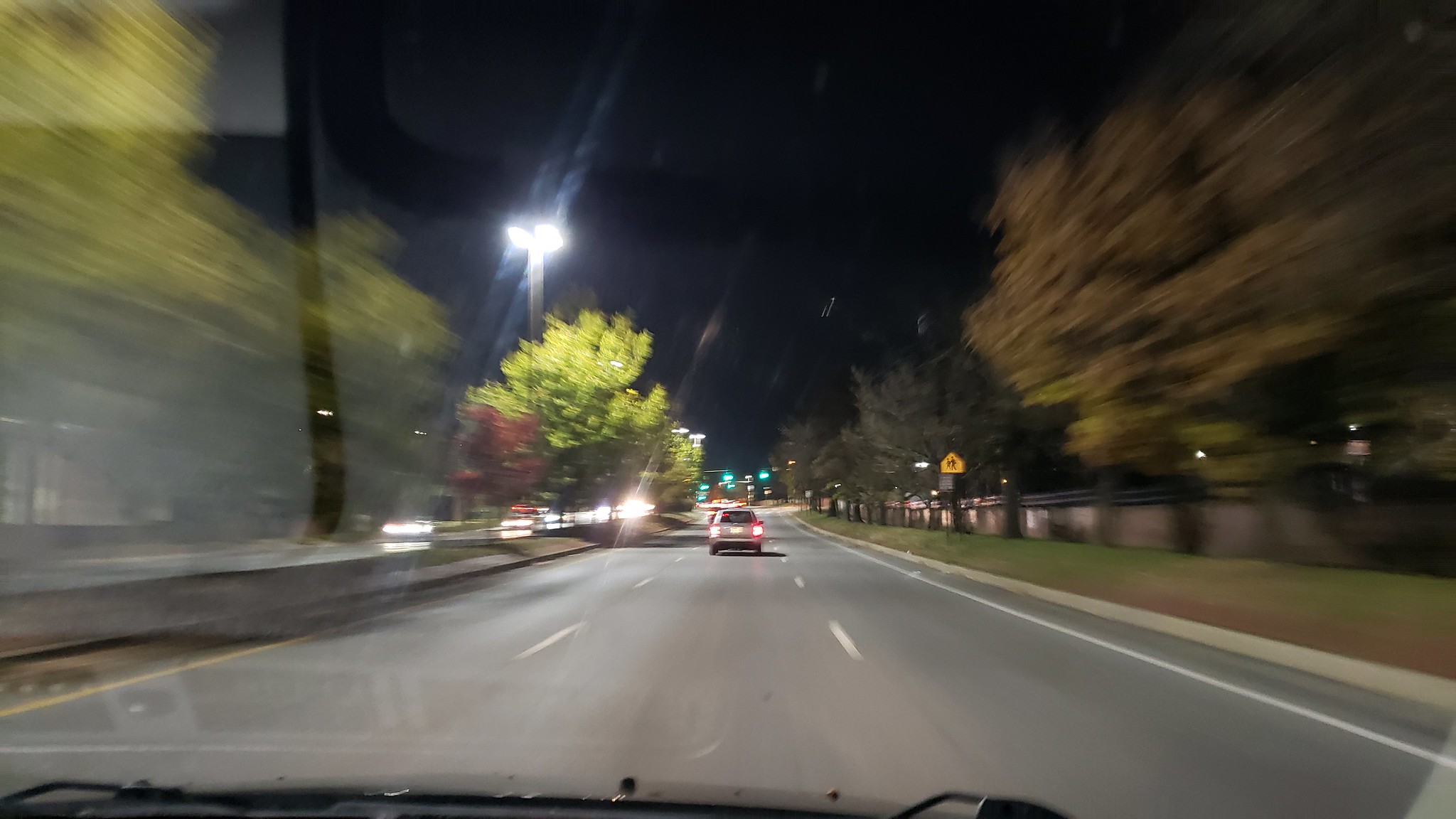This photograph, taken from the dashboard of a moving vehicle at nighttime, presents a detailed view of a three-lane road. The sky is solid black, indicating it is nighttime. Visible at the bottom are black windshield wipers. The long, gray road ahead features white dotted lines and a solid white line on the right. Green trees line both sides of the street, interspersed with residential houses partially obscured by a tall, built-up wall, likely made of brick or stone. The houses reveal small glimmers of lights through their windows.

A yellow pedestrian crossing sign, denoting a school crossing zone, is visible. Farther ahead, a traffic light emits a green signal, approximately half a mile in the distance. The scene also captures a bright street lamp on the left side, illuminating the road. The car directly in front has its red taillights on, and on the opposite side of the street, headlights of oncoming cars are visible, hinting at a busy six-lane thoroughfare. The image, though slightly blurred, conveys a vivid nighttime roadscape.